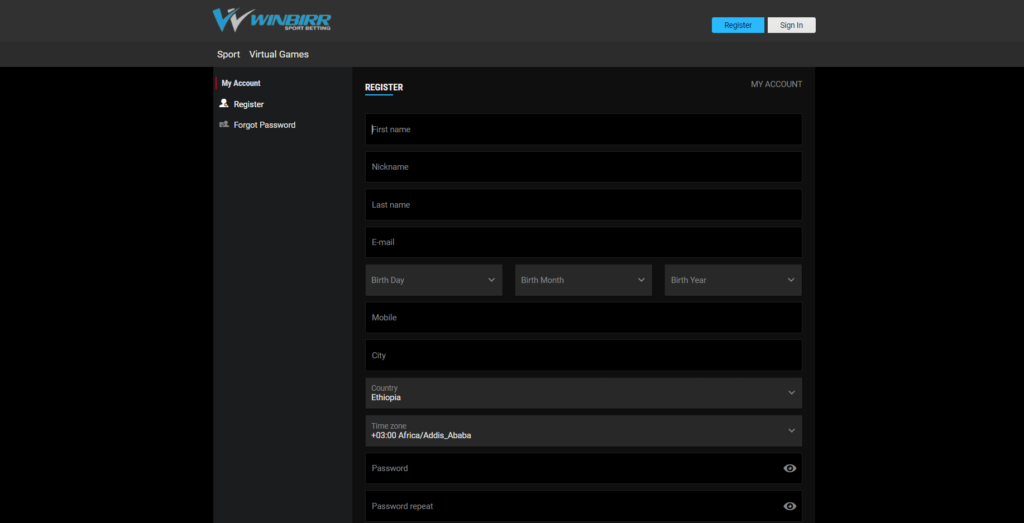This screen-captured image is of a website named WinBurr—spelled W-I-N-B-I-R-R—which is dedicated to sports betting. The WinBurr logo features a stylized "W" composed of two intersecting "V" shapes; the left "V" is teal and the right one is white.

At the top of the webpage, there is a user interface panel with a prominent blue button labeled "Register" and a white button labeled "Sign In." Directly beneath the WinBurr logo, categories such as “Sport” and “Virtual Games” are listed. 

On the same line, there is a section titled "My Account," marked by a vertical red line for emphasis. This area also includes links for "Register" and "Forgot Password."

The central part of the image displays a registration form with fields for personal details, arranged in a structured manner. The fields include "First Name," "Nickname," "Last Name," and "Email." There are also dropdown menus for entering your "Birthday," "Birth Month," and "Birth Year." Additional fields require information such as "Mobile," "City," "Country," "Time Zone," "Password," and a confirmation field labeled "Password Repeat."